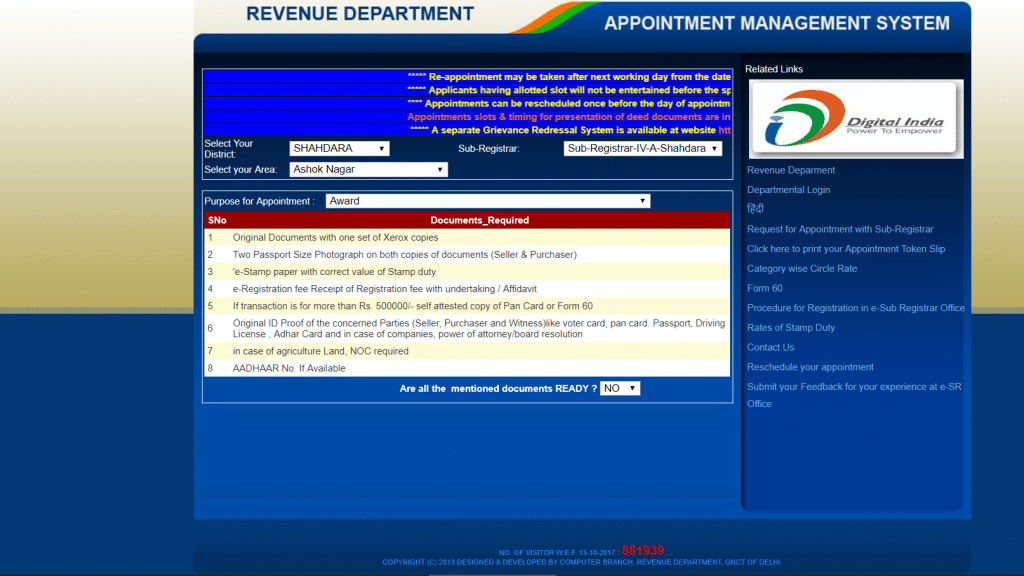The image displays the homepage of a government-run website in India, specifically for the Revenue Department's Appointment Management System. The design is predominantly blue, accented with vibrant shades of orange, green, yellow, and red, giving it a colorful, retro 90s aesthetic. Notably, the page features the "Digital India" logo with the slogan "Power to Empower".

There are various sections on the homepage, each enclosed in distinctive blue boxes. One of the notices reads: "Reappointment may be taken after the next working day from the date..." followed by text obscured by multiple asterisks. Similarly, another notice states: "Applicants having allotted slots will not be entertained before the..." with additional information also hidden by asterisks. Another key notice highlighted in red informs users, "Appointment slots and timing for presentation of documents are...," indicating specific instructions for document submissions.

The form includes dropdown menus for selecting various options. For instance:
- "Select your District": Shahdara was selected.
- "Sub-Registrar": Sub-Registrar 4VA Shahdara was selected.
- "Select your Area": Ashok Nagar was chosen.

Additionally, there is a section labeled "Purpose for Appointment," where users can select from approximately eight different listed purposes. The interface, while functional, retains a nostalgic look reminiscent of older web design styles.